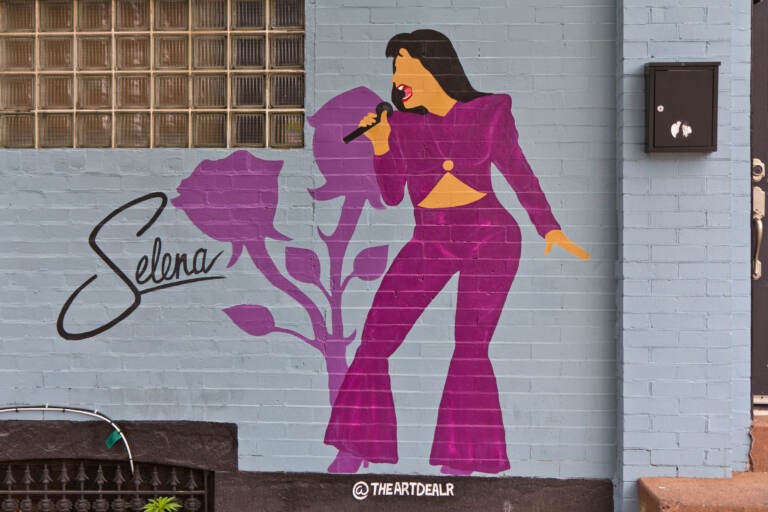This image captures the detailed mural of the famed Hispanic singer Selena on the side of a blue-toned gray brick building. The wall features a window of thick glass blocks that provide diffused light. Selena, depicted in a vivid purple outfit with long bell-bottom pants and a midriff-revealing blouse, stands prominently with her head facing left. Her long, dark black hair cascades to her shoulders, and light orange skin contrasts against the bold colors of her attire. Heavy shoulder pads and full-length sleeves accentuate her blouse. In her right hand, she holds a microphone close to her open mouth, highlighted by her red lipstick and teeth. The mural's background subtly shows the silhouette of two roses, casting shadows near her feet. To the left, Selena's name is written in black, pop star-style cursive, underlined for emphasis. The artwork is signed at the bottom with the artist's name, "The Art Dealer," accompanied by a circled 'A.' On the right side of the building, a black metal mailbox with a keyhole can be seen, adding to the scene's urban detail.